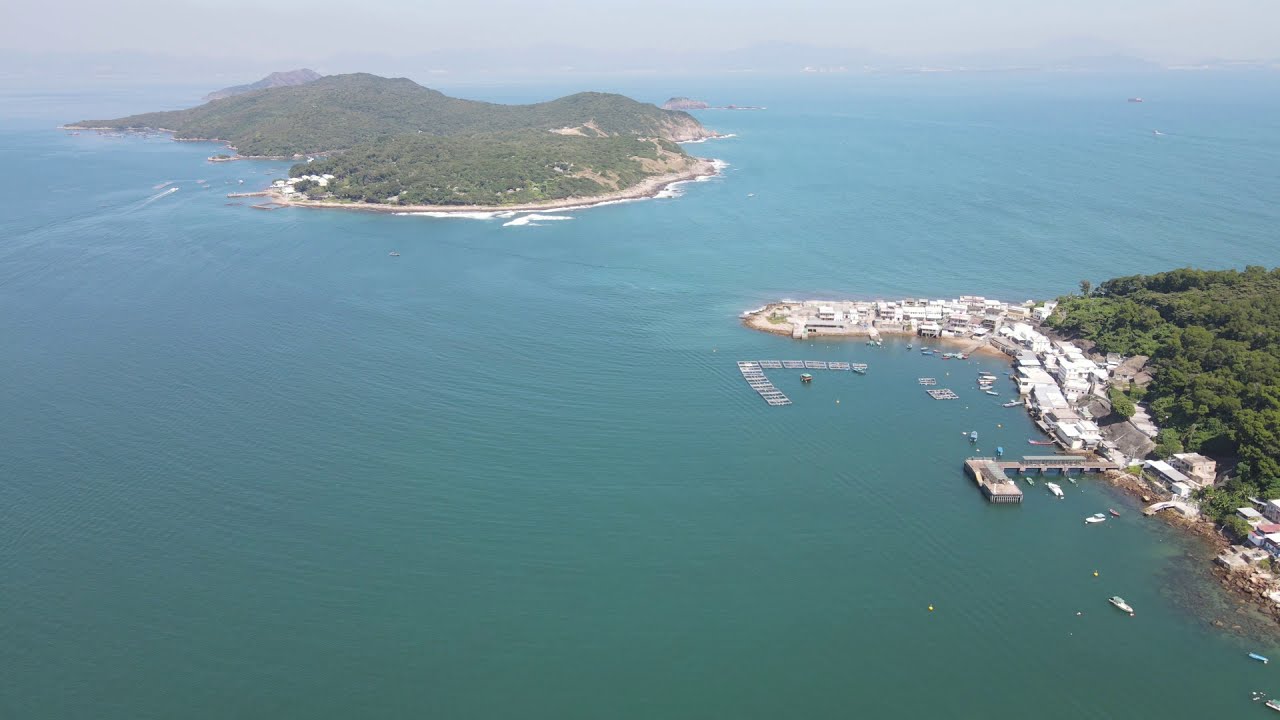The image is an expansive, overhead shot of a large body of water, likely an ocean or a massive lake, dominated by two major landmasses. In the upper left corner, there's a nearly circular island with jagged edges, featuring a light dirt-colored beach that darkens as it meets the water. The interior is densely covered in dark green trees. On the bottom right, another land section is visible, lush with thick trees on its right side. A peninsula juts into the water from this section, adorned with numerous buildings and bordered by docks extending into the water, some of which are occupied by white boats and jet skis. Close to the peninsula, there's a floating item resembling wooden pallets bolted together.

In the far background, the scene is enveloped in a hazy atmosphere, obscuring a distant row of mountains. The sky shares this haziness, blending seamlessly with the distant mountains. Scattered throughout the water are additional boats. The overall perspective suggests the photo was captured from a high vantage point, possibly from a drone or an airplane, emphasizing the vastness of the watery expanse, which constitutes about 60%-70% of the photo. The scene is picturesque, akin to a postcard, showcasing a serene yet bustling waterfront community.